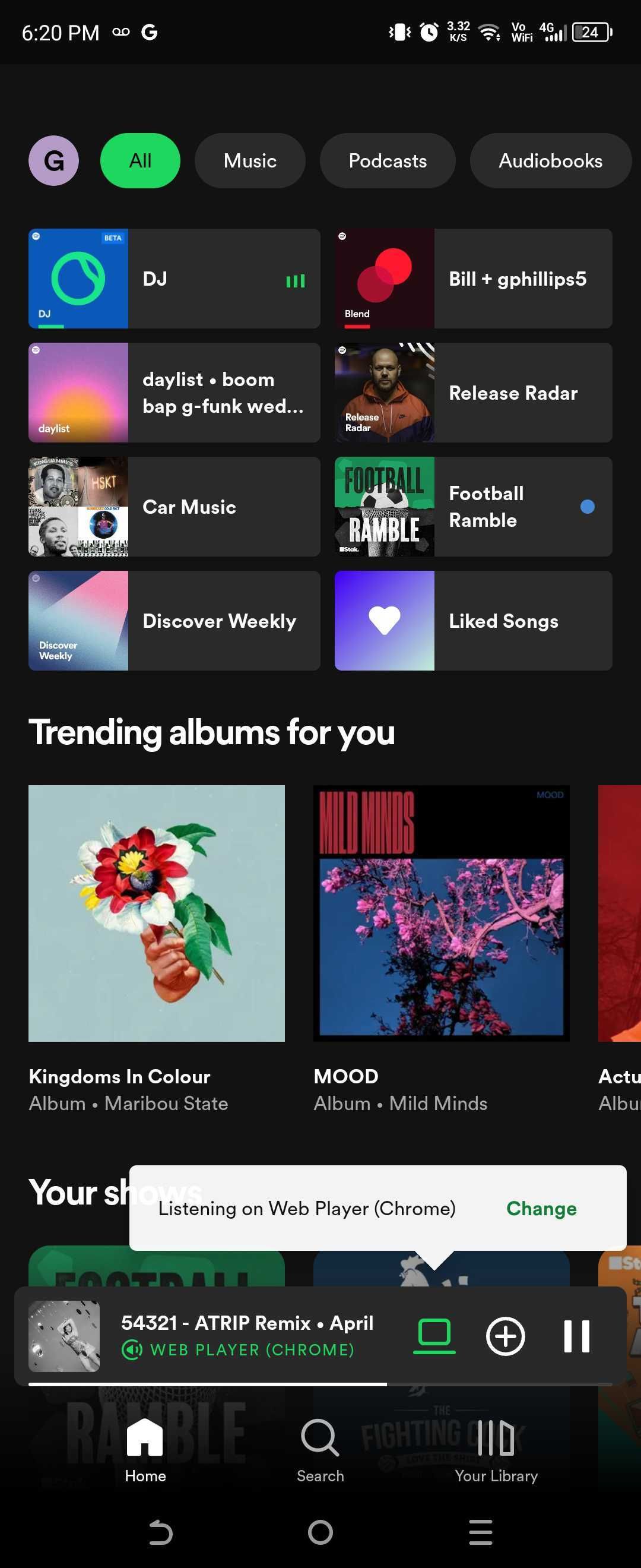The image appears to be a screenshot from a mobile phone. The background is black, and the text is white. In the upper left corner, the time reads "6:20 PM," and next to it is a Google icon. On the upper right are several mobile icons, including a battery indicator. 

Underneath, there is a grey circle with a 'G' inside, followed by a navigation bar with four options: "All," "Music," "Podcasts," and "Audiobooks." The "All" button is selected in green. Below this bar are four rows of content represented by sets of two squares each containing various symbols and images.

The top row features a blue circle with "DJ" written next to it. To its right are two red circles in a brown background, labelled "BIM," "BM," and "Gorillaz 5." Next to these is an icon showing a yellow sun against a pink sky and an image of a man's head with a distinct release pattern. The next visible icon is labeled "Car Music," featuring the heads of two people and an icon for "Football," which is a simple black and white illustration.

Further down is an icon for "Discover Weekly," with white text on a blue and pink gradient, and another called "Unlike Songs," represented by a white heart on a blue background. Below this section is a header that reads "Trending Albums for You," with a variety of album covers. One shows a red and white flower in grey, and another features an abstract blue and pink design.

On the side, there is text for "Kingdoms in Color" and "Mood." A white rectangle with black text at the bottom partially obscures additional content. Below this rectangle, it mentions "Listening on Web Player (Chrome)" with an option to "Change."

At the bottom of the screen is a grey icon with white writing that says "Five, Four, Three, Two, One," followed by abbreviations "A, T, R, P," and the phrase "Remix April," suggesting a currently playing song. Accompanying this is a green play button and a plus button to its right-hand side.

Lastly, the bottom of the screen displays navigation icons for "Home," "Search," "Your Library," with another "Back" button, a second "Home" button, and three horizontal lines indicating a menu.